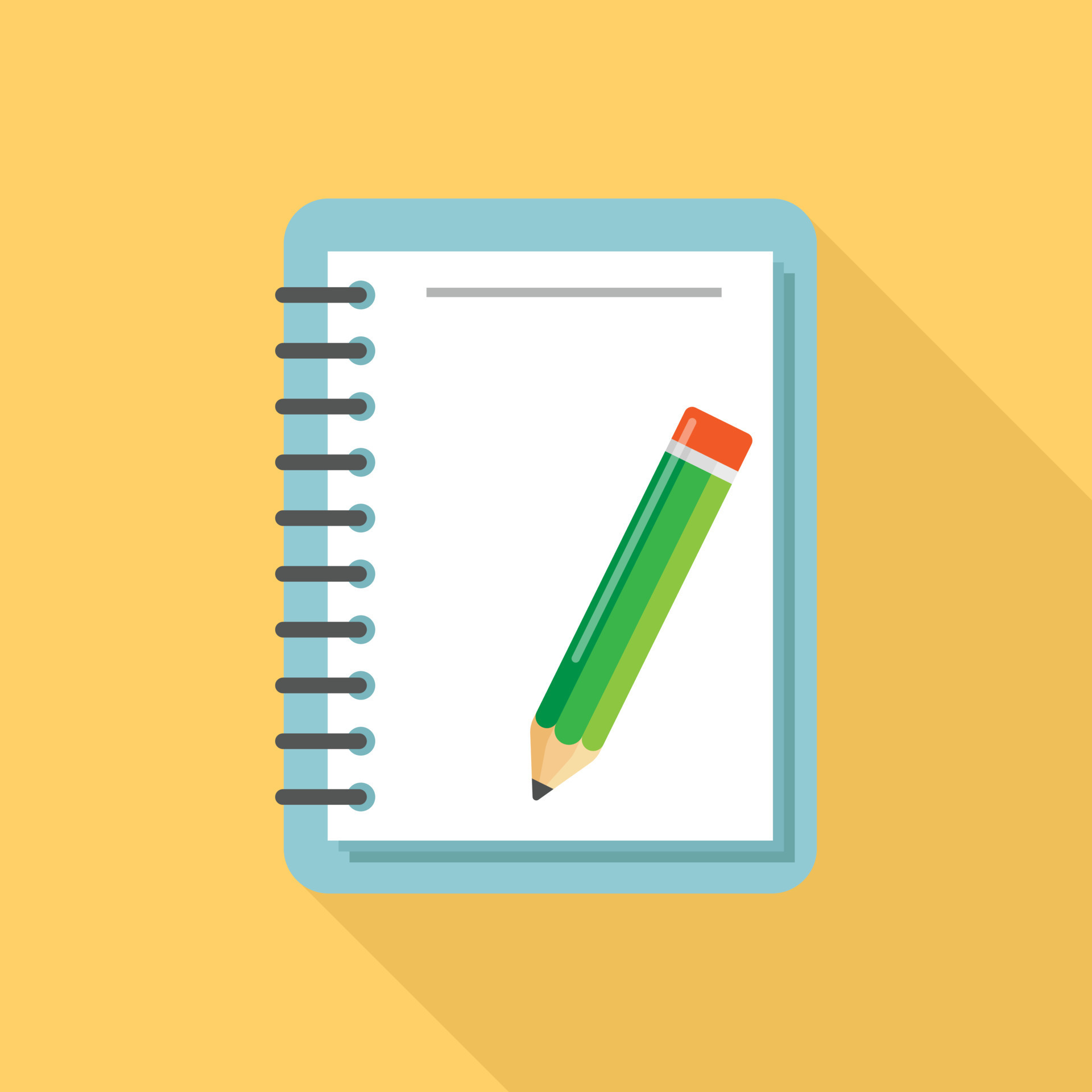The image is a graphic illustration featuring a notepad with dark gray ring binding on the left side and a cover in light blue. The notepad's paper is white with a small gray bar at the top. A green pencil with a typical pink eraser and sharp point is angled across the front of the notepad, pointing to the bottom left. The entire scene is set against a yellowish cream background, with the notepad casting a shadow that extends to the bottom right, suggesting that the light source is from the top left.